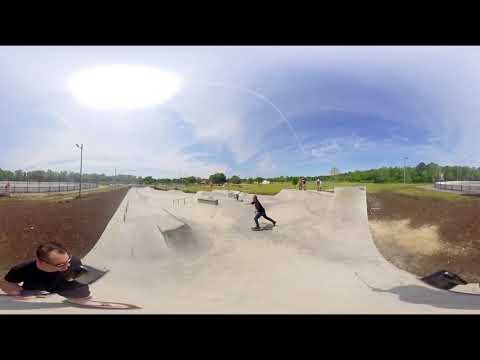The image captures an expansive, outdoor skate park on a bright, blue-skied day with scattered gray clouds. The central focus is a man skateboarding, dressed in a black shirt and black pants, mid-action in the park's concrete expanse, which features a half-pipe, rails, and other skating structures. The scene has a slight fisheye distortion, adding a unique perspective to the photograph. In the lower-left corner, a person with brown hair and glasses walks by, slightly distorted, emphasizing the fisheye effect. The park is bordered by a green grassy field with trees and light poles, along with visible power lines. A sandy patch surrounds parts of the skate park, and in the distance, a gray building and a fence are noticeable. The sunlight bathes the entire area, highlighting the vibrant activity of four or five skateboarders immersed in their tricks and interactions.